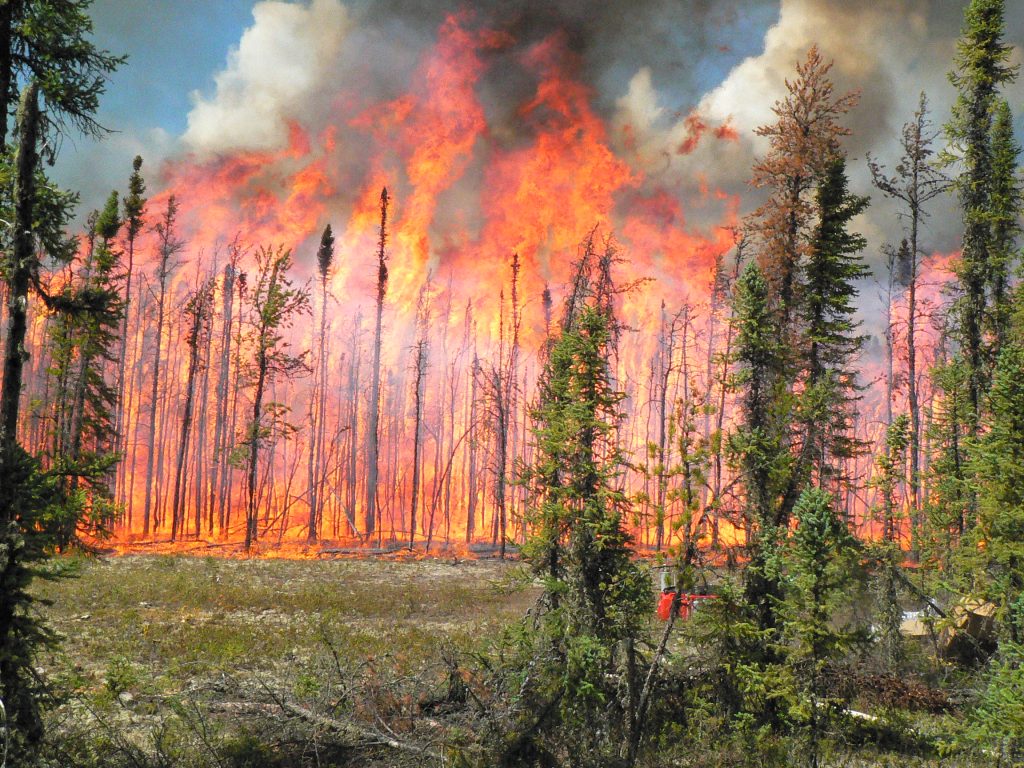The image captures the stark contrast of a forest fire's devastation. In the foreground, there's a tranquil stretch of flat land, characterized by short green grass and patches of whitish-grey sand. About half a dozen tall, thin trees stand intact with their green leaves or foliage still vibrant. To the right, there appears to be some scattered rubble, possibly including a red object and what looks like cardboard boxes.

In sharp contrast, the background is awash with the chaos of the fire. The fire itself is a fierce blaze, a mix of intense reddish and orange hues, consuming everything in its path. The trees there are stripped bare, reduced to blackened, barren trunks standing like ghostly silhouettes. Thick black smoke rises from the flames, mixing with the clouds above against a backdrop of blue sky, highlighting the destructive power of the wildfire. The entire scene vividly captures the moment, balancing the untouched serenity of the foreground with the fiery devastation behind.